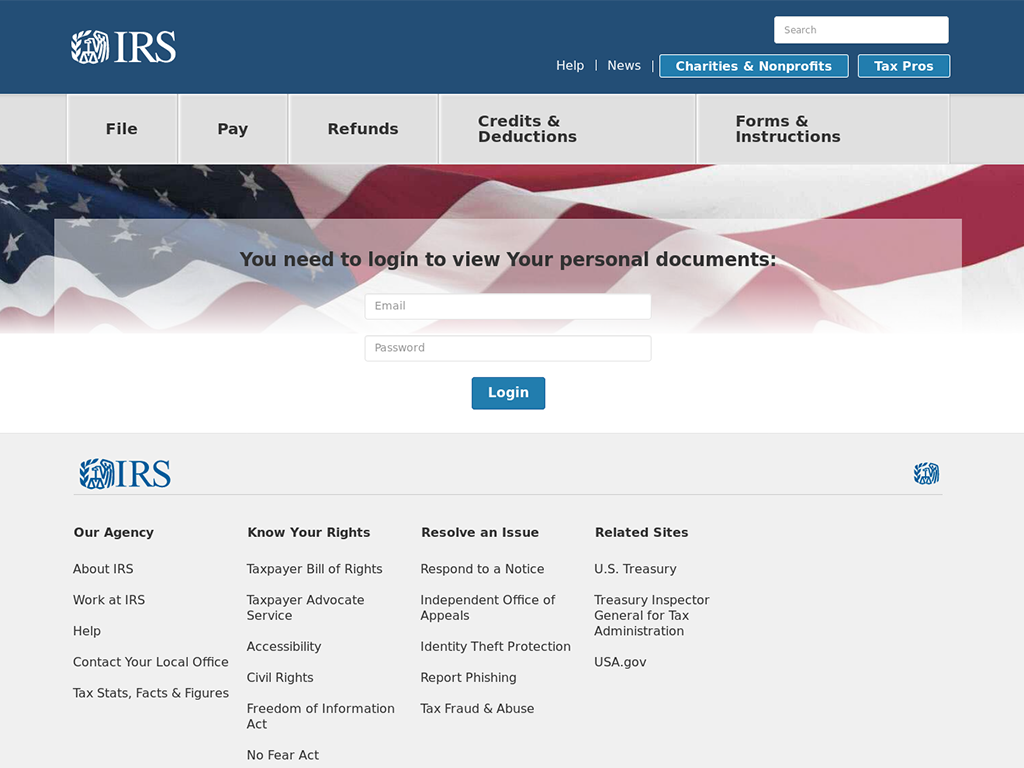The image captures a screenshot of the IRS website. At the top is a blue banner featuring the white IRS logo, which includes an eagle with a laurel leaf. Alongside it is a white search box and navigation links labeled "Help," "News," "Charities and Nonprofits," and "Tax Pros" in blue and white.

Below this main navigation, there are gray and black submenus with categories such as "File," "Pay," "Refunds," "Credits and Deductions," and "Forms and Instructions."

Prominently displayed in the center of the page is a white box with black text stating, "You need to log in to view your personal documents." This section includes fields to enter your email and password, along with a blue and white login button. The backdrop of this section features an American flag in red, white, and blue.

At the bottom of the screenshot, a gray footer contains the IRS logo and various submenus, including "Our Agency," "About IRS," "Work at IRS," "Help," "Contact Your Local Office," "Tax Stats," "Facts and Figures," "Know Your Rights," "Taxpayer Bill of Rights," "Taxpayer Advocate Service," "Accessibility," "Civil Rights," "Freedom of Information Act," and "No Fear Act." It also provides links under "Resolve an Issue" such as "Respond to a Notice," "Independent Office of Appeals," "Identity Theft Protection," "Report Phishing," "Tax Fraud, and Abuse."

Additionally, there are sections labeled "Related Sites" with links to "U.S. Treasury," "Treasury Inspector General for Tax Administration," and "USA.gov." Another eagle and laurel leaf symbol is situated towards the bottom right of the image. The overall image is very clear with bold, easy-to-read font, free of any pixelation or blurring.